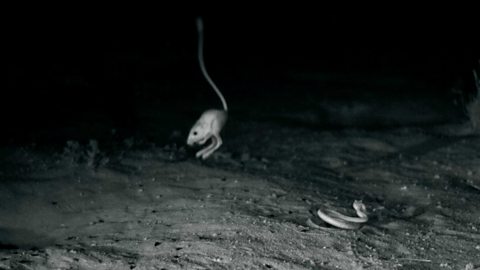This black-and-white night vision photograph captures an intense nocturnal scene in a sandy, desert-like environment dotted with small rocks and pebbles. At the heart of the image is a kangaroo mouse, dramatically suspended mid-jump, its body lit stark white against the pitch-black background. The mouse's long, L-shaped hind legs are clearly visible, emphasizing its kangaroo-like appearance, while its exceptionally long, thin tail arches high into the air, almost resembling a worm. In the bottom right corner, a snake is coiled and poised to strike, adding a palpable sense of danger to the scene. The ground is textured with dirt and sparse vegetation, and the overall setting hints at a dry, arid landscape. The contrasting elements and the frozen motion of the kangaroo mouse create a captivating, dynamic snapshot of nocturnal wildlife.